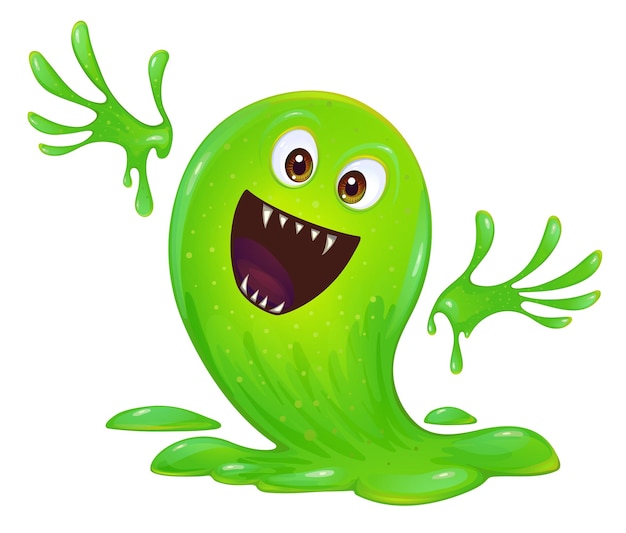In this digital artwork, we see a friendly green slime monster, whimsically shaped like a ghost or teardrop, with a bright, shiny green hue. The bottom of its form spills out onto the floor, creating small green puddles of slime. Floating beside its body are two unattached, dripping green hands, adding to its quirky appearance. The monster has large, expressive eyes with whites resembling eggs and prominent brown irises, which give it a friendly demeanor. Its wide-open mouth, set in a broad smile, reveals sharp white teeth—five on the top and four on the bottom—making it look both endearing and mischievous. The entire scene is set against a plain white background, allowing the colorful, playful details of the monster to stand out.